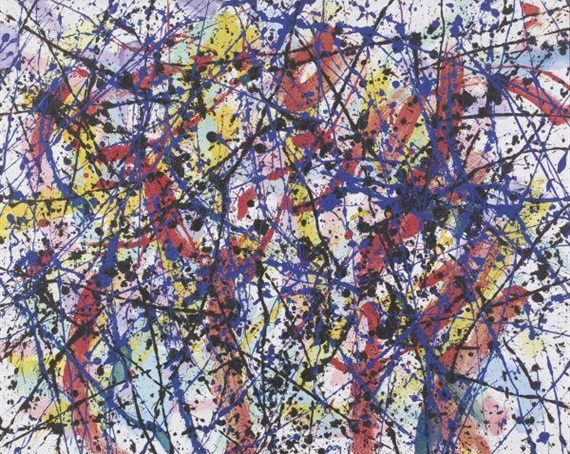The image depicts an abstract painting on a light-colored or off-white canvas. Dominated by an array of vibrant paint streaks and splatters, the painting features thick red and yellow lines that criss-cross across the canvas, creating a chaotic but compelling design. These bold streaks almost resemble text but remain ambiguous. Over these prominent lines, layers of black, blue, and purple paint have been splattered, with blue and black forming both streaks and dots, while purple tends to appear as linear splatters. The paint extends all the way to the edges of the canvas, which is unframed, giving it a raw and unbounded aesthetic. The composition concludes with splatters and smudges scattered throughout, adding layers of complexity and texture to the painting.